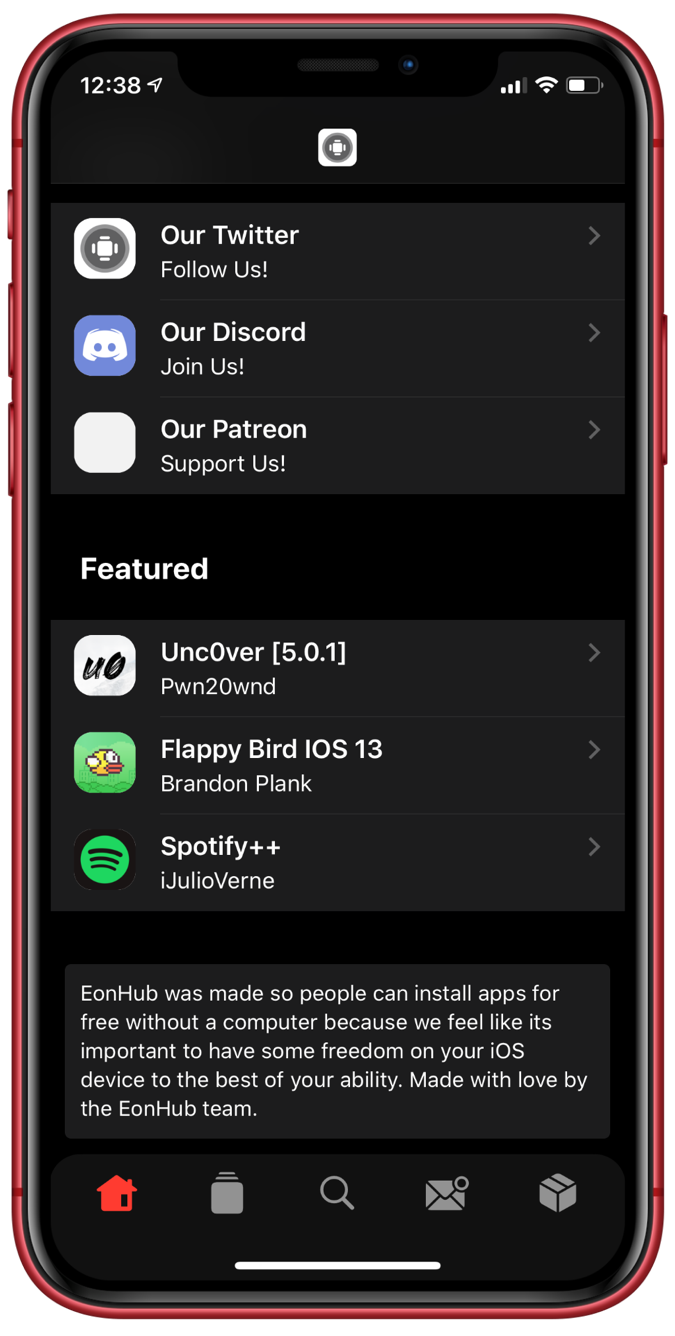A detailed image caption that is cleaned up and formulated could be:

"A black smartphone with a red case is lying on a surface. The phone has three red buttons on the left side and one red button on the right side. The screen is black, displaying the time '12:38' in white text at the top left corner. Next to the time, there is a white arrow pointing to the right, followed by a small blue dot. The signal indicator shows three white bars and one dark gray bar, indicating partial signal strength. The Wi-Fi icon is fully filled and next to it, the battery icon indicates a little over 50% charge in white. Below this, there is a white square icon containing a gray circle, and within the gray circle, there is a white rectangle with dashes on either side. Further down the screen, text reads 'The White Hour: Twitter - Follow Us!', 'Our Discord - Join Us!', 'Our Patreon - Support Us!'. It also lists several app features including 'Uncover 5.0.10', 'PWN20', 'WND', 'Flappy Birds', 'iOS 13', 'Brandon Blanks', 'Spotify++', and 'iJulio Verne'."